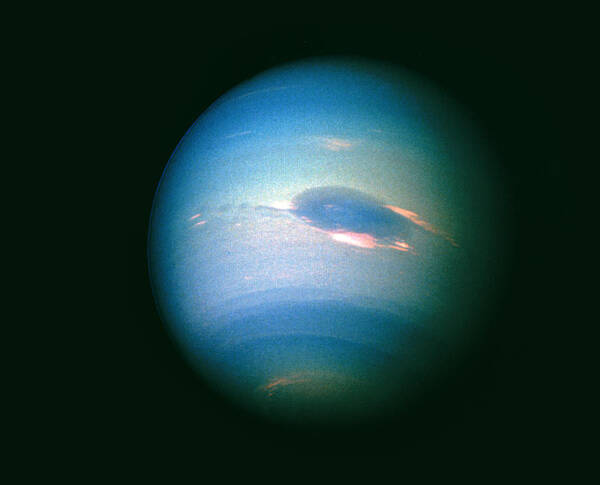The image features a blue planet surrounded by the vast blackness of space, its left side illuminated by a light source, while its right side fades into darkness. The planet's surface showcases various shades of blue, predominantly a deep oceanic hue, interspersed with streaks of white. The central part of the planet features a dark blue spot, reminiscent of a swirl, with a haze of white enveloping it. There is also a long arm of light blue extending from this swirl, curving gracefully around the planet. This arm is accompanied by smears of white on both the top and bottom. Additionally, the bottom of the planet displays a lighter color with another darker blue swirl within it. The entire scene, possibly a photograph or an artistic representation, appears slightly blurry, evoking a vintage or old-school aesthetic. The planet's appearance hints at it being a gas giant, though its true identity remains uncertain, with its coloration reminiscent of Pluto.